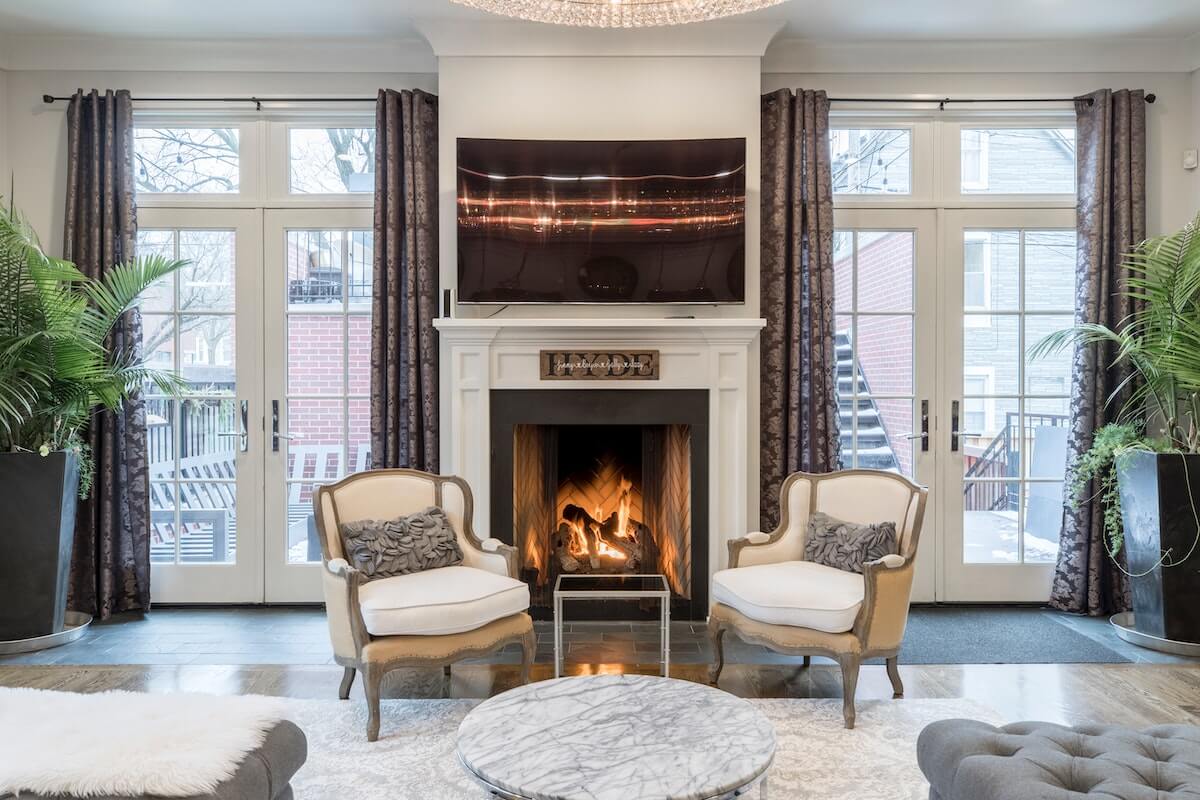The photograph captures a meticulously symmetrical living room, centered around a lit fireplace topped by a flat-screen TV. The TV screen displays what appears to be the reflection of city lights, adding a dynamic focal point above the fireplace, which bears a sign reading "HIDE." Flanking the fireplace are double French doors with transom windows above, draped with brownish metallic curtains that are pulled open to reveal daylight outside. 

In front of the fireplace, two elegant armchairs with beige upholstery and gray rectangular pillows stand, separated by a small coffee table. These chairs feature prominent white cushions and ornate wood trim. A round marble-topped table occupies the middle of the room, complemented by two tufted gray ottomans positioned on either side. One ottoman is plain gray, while the other is adorned with a faux white fur cover. Completing the scene, tall square planters with lush greenery are placed near the windows.

The overall ambiance is one of refined elegance, combining cozy elements like the lit fireplace and plush seating with sophisticated decor and a harmonious layout.